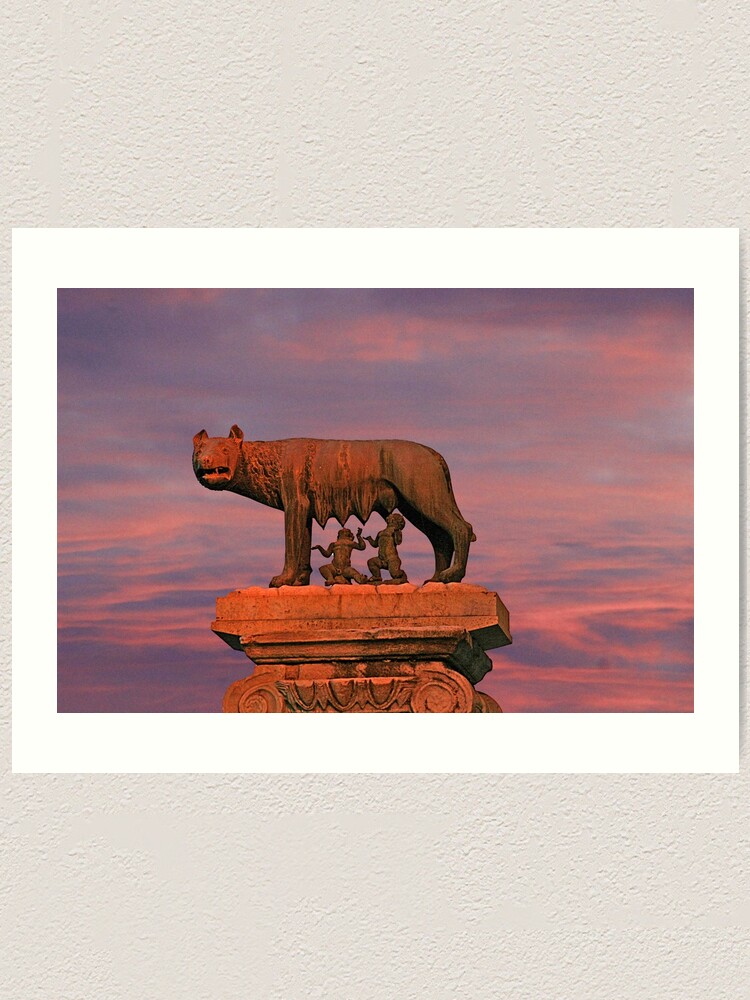The image is a photorealistic postcard displayed on a white wall. It features a statue of a wolf with pronounced teats on top of a stone pillar, bathed in an orange light. The statue, likely representing the Roman myth of Romulus and Remus, depicts two small boys suckling at the wolf's teats. The background showcases a vibrant sky at sunset, colored in hues of blue, purple, pink, and magenta. The wolf's face is turned towards the camera, adding a lifelike quality to the postcard.